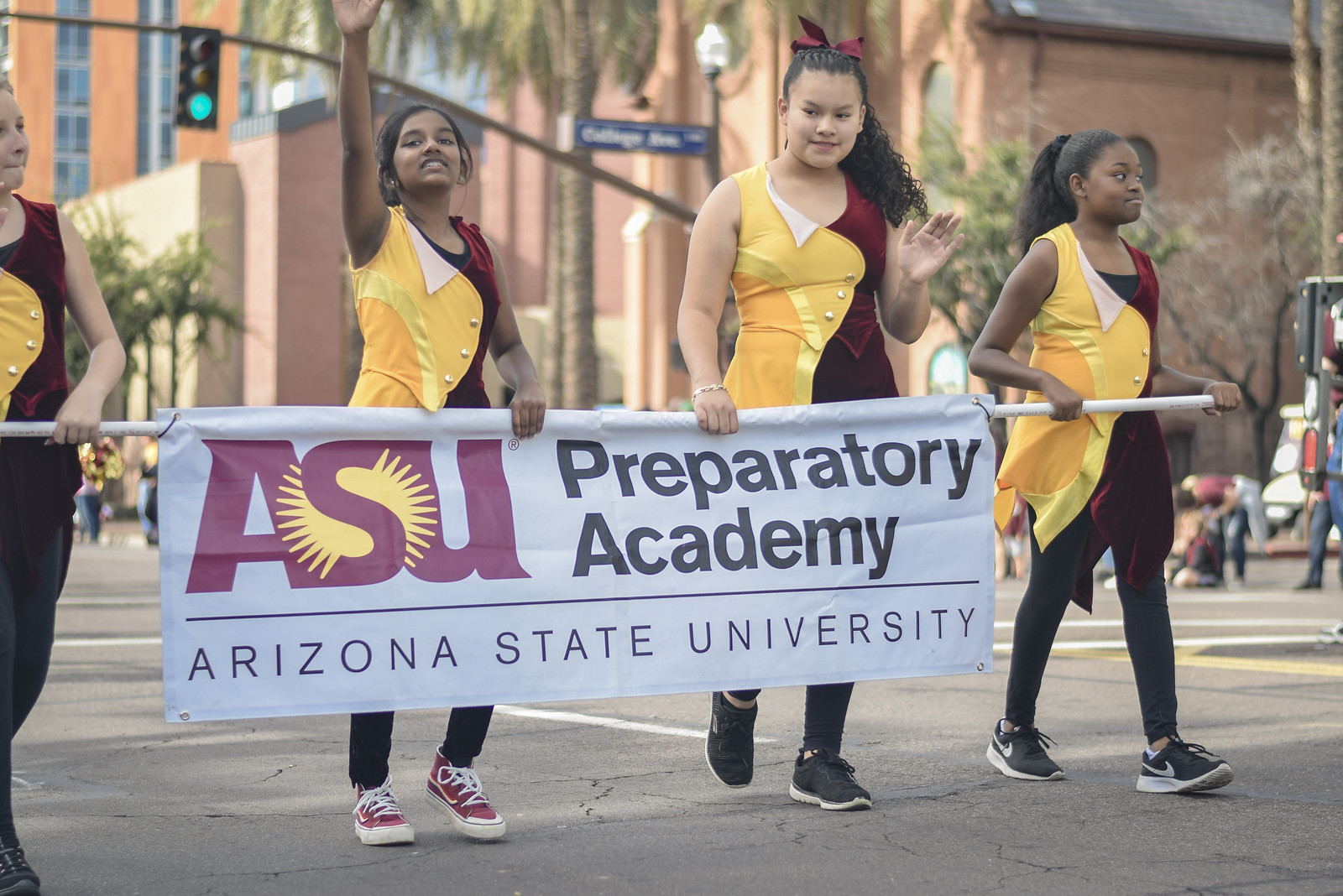In this vibrant color photograph, a parade unfolds down an asphalt street featuring four young women, who appear to be in their high school or early college years. Dressed in striking yellow and maroon marching band uniforms, paired with black pants or leggings and various colored sneakers, they stride in unison at the head of the procession. The girls are holding a white banner, hooked to a horizontal pole, which prominently showcases the text "ASU" with a stylized sun behind the "S", and further reads "Preparatory Academy" followed by "Arizona State University" in bold black text. The background reveals a bustling scene with a mix of participants and onlookers, an orange brick building with windows, a green-lit traffic signal, and a blue street sign marked "College Avenue" attached to a light post. The photograph captures the lively spirit and structured formation typical of a parade, punctuated by these vivid details and harmonized colors.